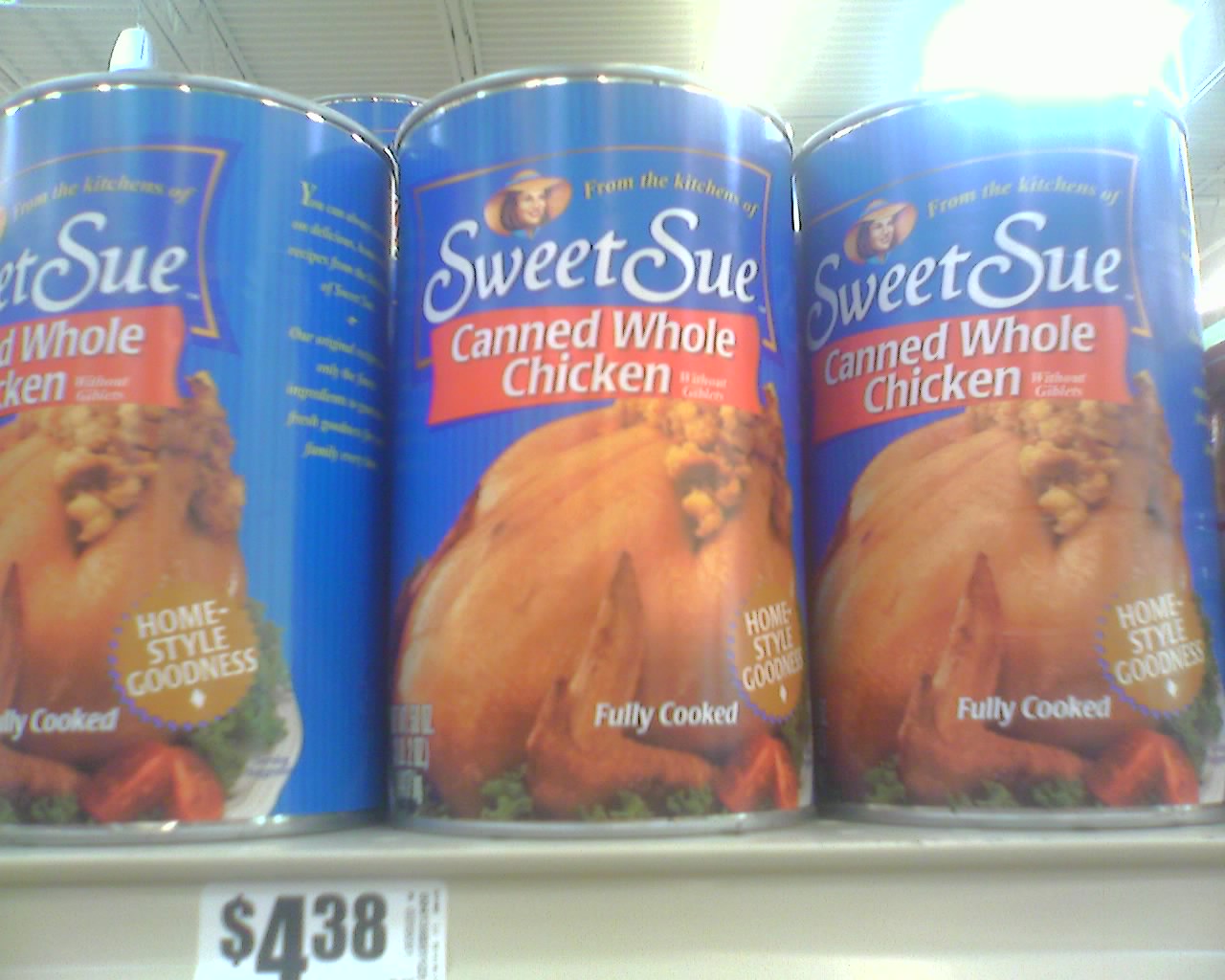This photograph, taken inside a store, captures a shelf displaying three cans of Sweet Sue canned whole chicken, priced at $4.38 each. Despite the blurry and low-quality nature of the image due to a smudgy camera lens, several details are discernible. The tops of the image feature two rectangular lights emitting a bright bloom effect and the white roof of the building which has a blind-like appearance with horizontal grooves. The cream-colored plastic shelf, located at the bottom, holds the cans prominently.

Each blue-labeled can of Sweet Sue showcases a white-font title and beneath it, a graphic of a white woman with brown hair and a wide-brimmed hat, accompanied by the words "From the Kitchen of." Below the name Sweet Sue, a red bar with white text displays "Canned Whole Chicken," followed by a detailed photograph of a cooked chicken with a garnish of lettuce, and possibly a tomato or strawberry. The chicken appears fully cooked with a crisp skin, and the stuffing is visible, seemingly oozing from the bird. Additional text on the cans includes a white-font message "Fully Cooked" over the image of the chicken, as well as a red star proclaiming "Home Style Goodness." The shelf tag on the bottom left corner specifies the price in black text on a white background.